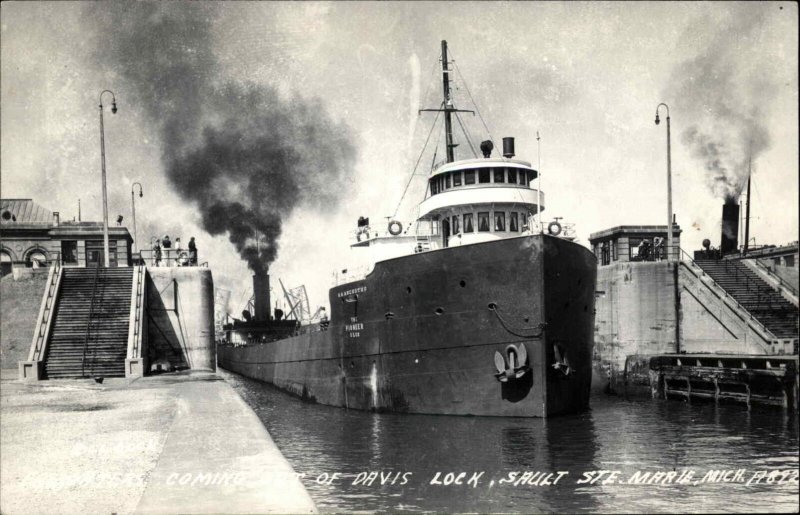This black and white photograph captures a historical scene at Davis Lock, Salt Ste. Marie, Michigan. The primary focus is on a large steamboat docked at the lock, emitting dark smoke from its tall smokestack. The steamboat's body appears dark with lighter upper structures, and a timestamp at the bottom right corner suggests it dates back to 1822 or 1892. 

In the foreground, several people stand on a concrete plateau to the left, accessible by stairs and adorned with curved streetlights. Another dock with stairs and a second steamboat with a smokestack is visible to the right. The photograph features a slightly wavy water surface and an overcast, grayish-white sky. Notably, there is white text at the bottom of the image providing information about the location and vessel, partially readable as "Davis Lock, Salt Ste. Marie, Michigan," though some details are obscured due to the light background.